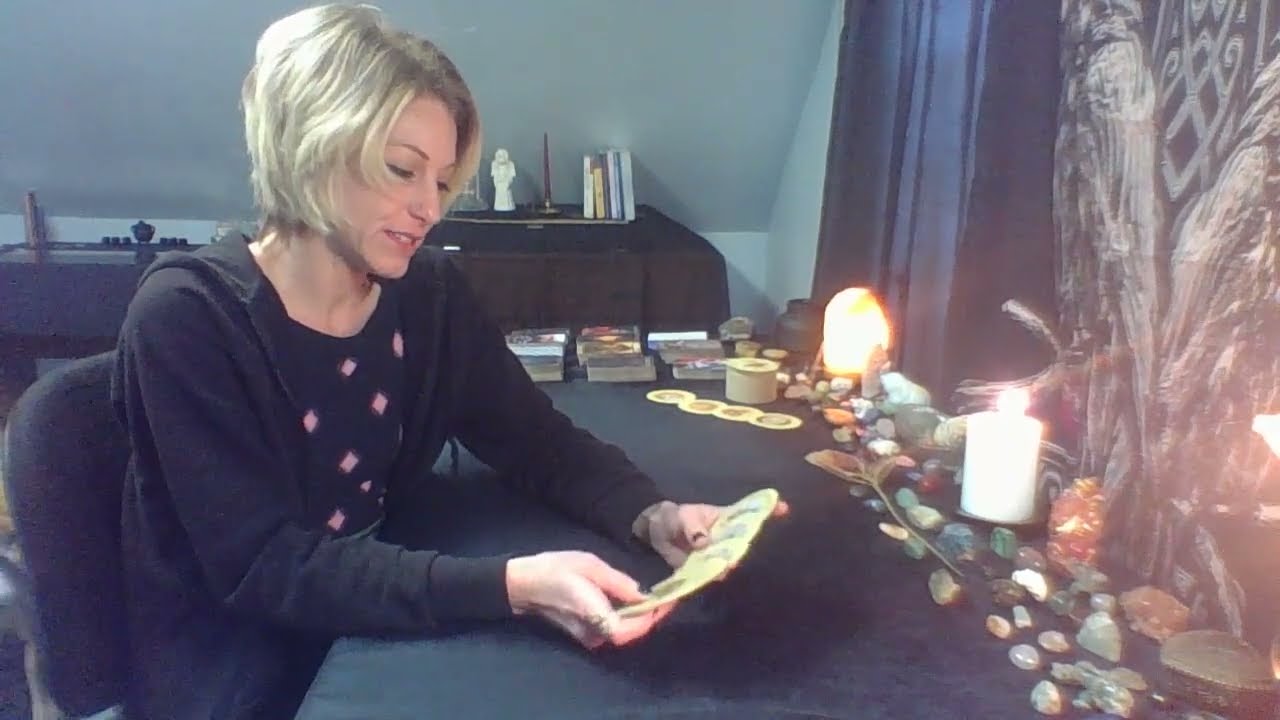The image captures a Caucasian woman, likely a fortune teller or spiritualist, engaged in a tarot card reading. She is seated in a black office chair at a dark-colored desk, looking down at an array of circular cards held in her extended hands. She has a distinctive "Karen" style haircut: short at the back in a pixie cut with longer sections at the front, parted slightly off-center. Her short blonde hair frames her face, which features very skinny tweezed eyebrows and light pink lip balm. She is dressed in a black hoodie over a black t-shirt adorned with a random assortment of pink diamonds.

The desk in front of her is scattered with multicolored healing stones, including opals, aventurine, labradorite, amethysts, and rose quartz. On the far left of the desk are stacks of tarot or card decks and possibly books. A lit candle flickers in front of her, adding a warm glow to the scene. 

The background of the image includes a blue slanted wall, suggesting she is in an upper-level room. Blue curtains drape on the right side, alongside a tapestry or poster with two ravens standing back-to-back on a branch against a backdrop with potential Celtic designs. Additional elements in the room include small statues, a stack of books, and another candle, contributing to an ambiance filled with mystical and spiritual décor.